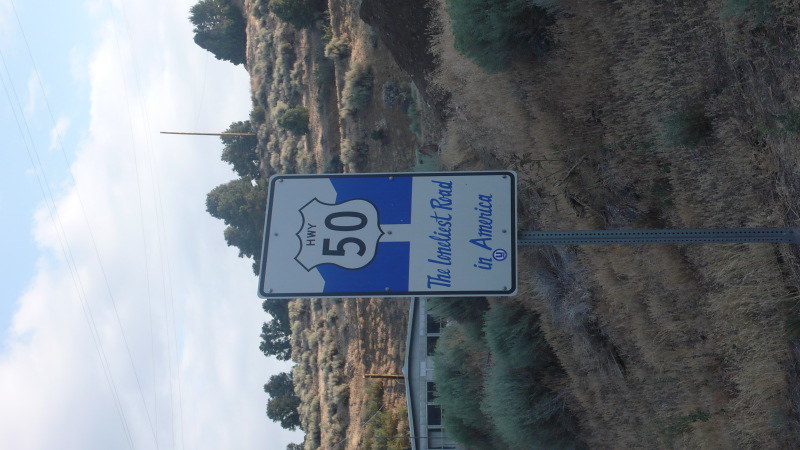The image depicts a sign, displayed sideways, that reads "The Loneliest Road in America" at the bottom and "Highway 50" at the top. The sign features a design reminiscent of a police badge, with "Highway" written in small letters at the top and "50" in large letters in the middle. The sign has a blue foreground and a white background with blue writing at the bottom. The scene appears to be set in a desert-like area, characterized by dry, brown vegetation and sparse greenery. In the background, there is a small house-like structure. The highway itself is not visible in the image, suggesting it was cropped out of the frame.